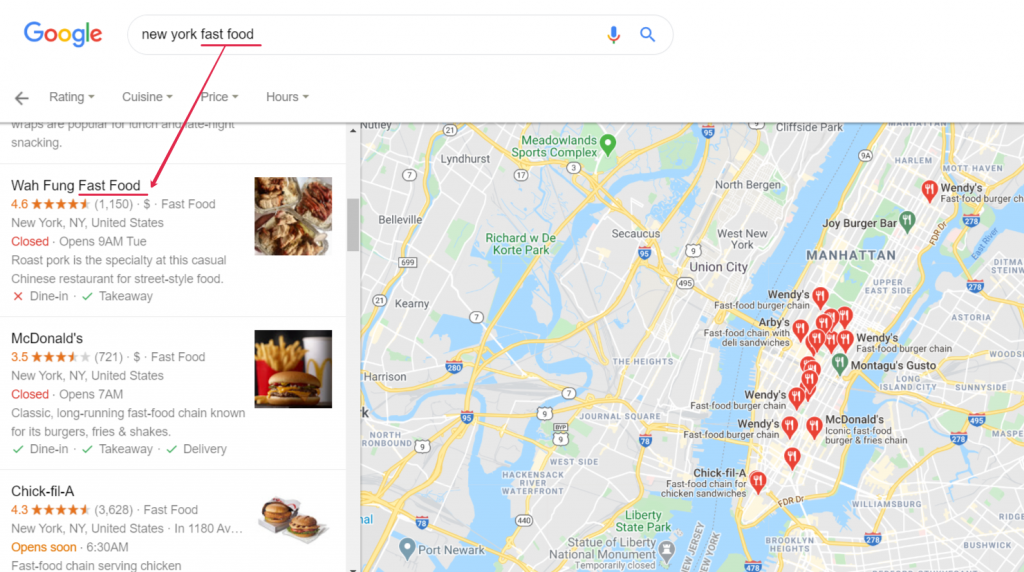The image displays a screenshot of a Google search map for "New York fast food," highlighting the search results and locations of several fast-food restaurants. The term "fast food" is underlined in two places, with a red arrow linking the search term at the top to the relevant results below.

Three featured restaurants are listed, starting with Wa Fung Fast Food, described as a casual Chinese restaurant known for its roast pork street food. It is marked as closed, with opening hours at 9 a.m. on Tuesday, and has a high rating of 4.6. An image of their food appears to the right.

Next is McDonald's, described as a classic long-running fast food chain famous for its burgers, fries, and shakes, with a corresponding picture of a McDonald's meal. This chain has a rating of 3.5.

Following that, Chick-fil-A is mentioned as a fast-food chain serving chicken, with a rating of 4.3. No image accompanies this entry.

On the right side of the image, a map of New York is shown with numerous pins—colored either red or green—indicating the locations of various fast-food establishments.